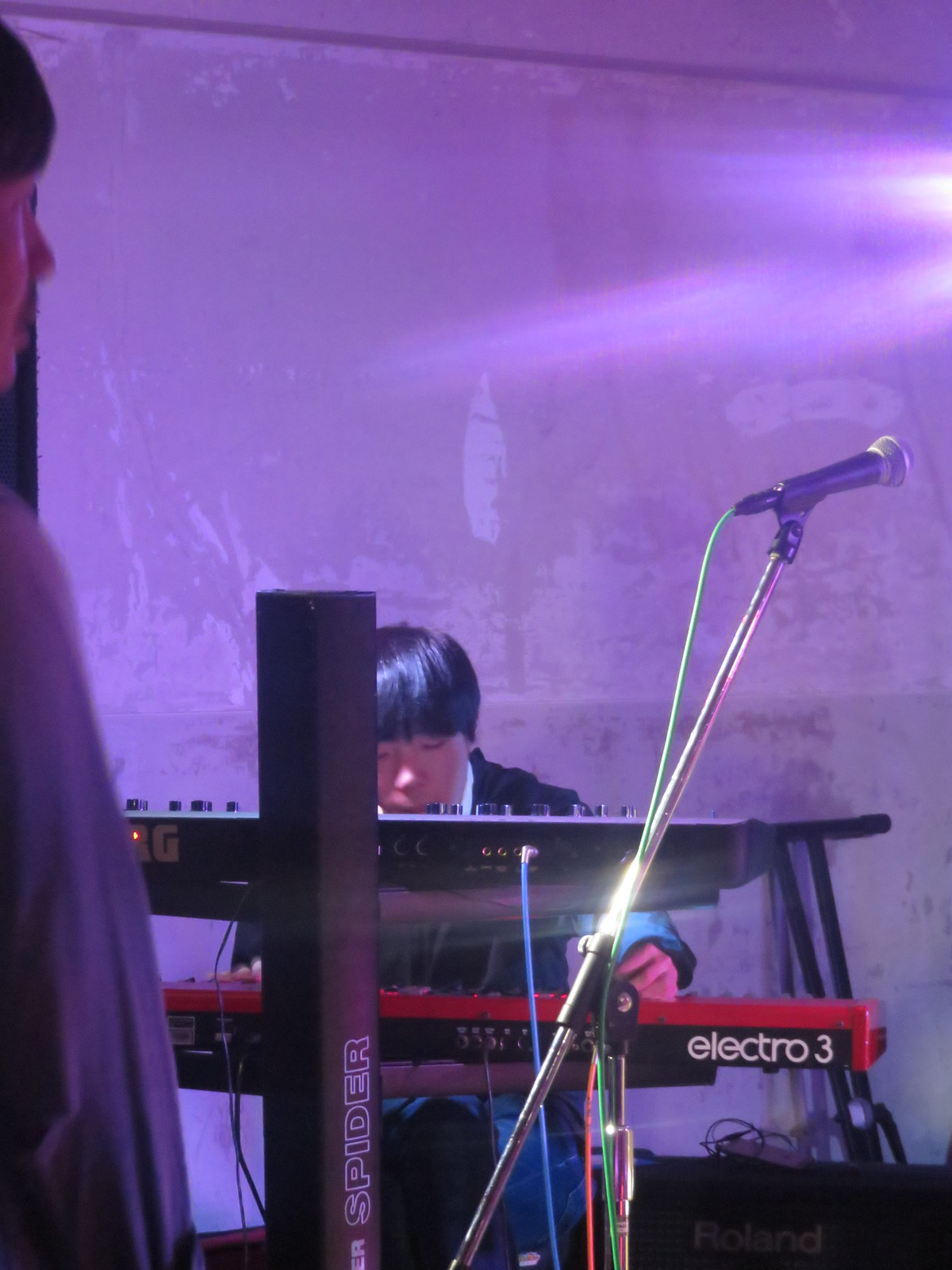In this vertically aligned rectangular image, we see a young man of Asian descent sitting at the center, playing two stacked electric keyboards with closed eyes, creating a focused atmosphere. He has short black hair in a bowl cut style and is dressed in a black shirt and pants. The image's background is dominated by a walled surface bathed in a purplish hue from the lighting, contributing to the overall stage effect.

On the left of the image, partially visible, is another man with short black hair, wearing a long-sleeved shirt, only his right shoulder and part of his face are seen. A gray pole labeled "Spider" stands prominently in the foreground, supporting the two keyboards. The upper keyboard is black with the text "Electro 3" in white letters, while the lower one has a red and black color scheme and a blue cord emerging from it. A black and gray microphone attached to a stand with green and orange cords extends towards the middle right, facing rightwards. Nearby, on the floor beside the man, there is a black square object marked "Roland." The detailed arrangement and color of the objects, along with the subdued lighting, create a vivid and dynamic depiction of a musical performance.